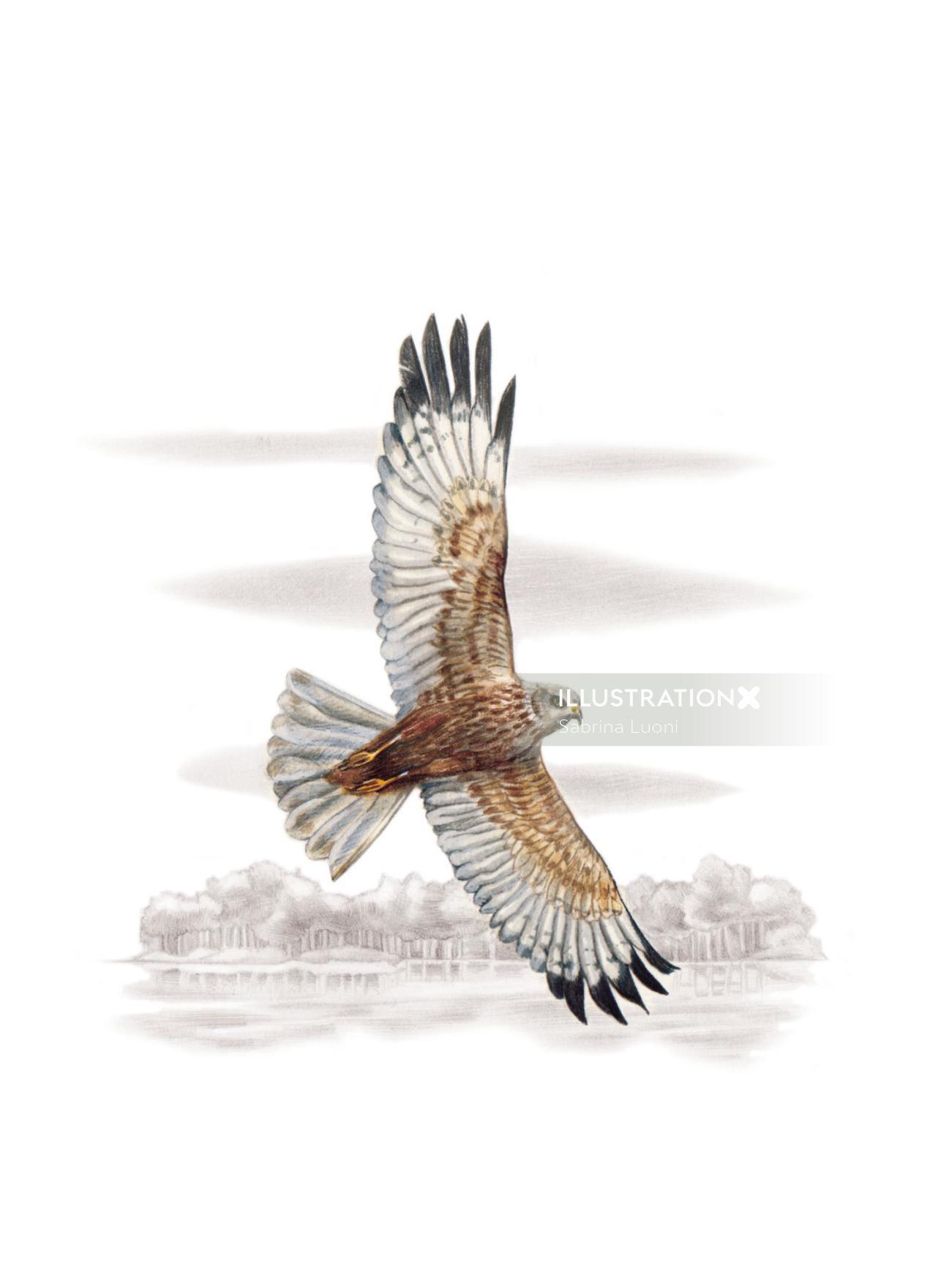The image is of an artwork titled "Illustration X" by Sabrina Luani, spelled L-U-A-N-I, with the text written in white near the top of the image. The piece captures a hawk in mid-flight, its wings fully extended with one wing facing the ground and the other the sky. The bird’s body is predominantly brown, with brown feathers on the upper part of the wings and black tips at the ends. The underside of the wings and the tail feathers are white, with the tail feathers fanned out in a display. Its legs are pulled close to its body, prominently yellow against the rest of its plumage. The background features a monochromatic landscape with softly rounded trees extending along a lakeshore, the water and land rendered in grayscale hues. The sky shows gray, streaky clouds, blending seamlessly with the subdued scene, making the vividly colored hawk the central focus of the artwork.